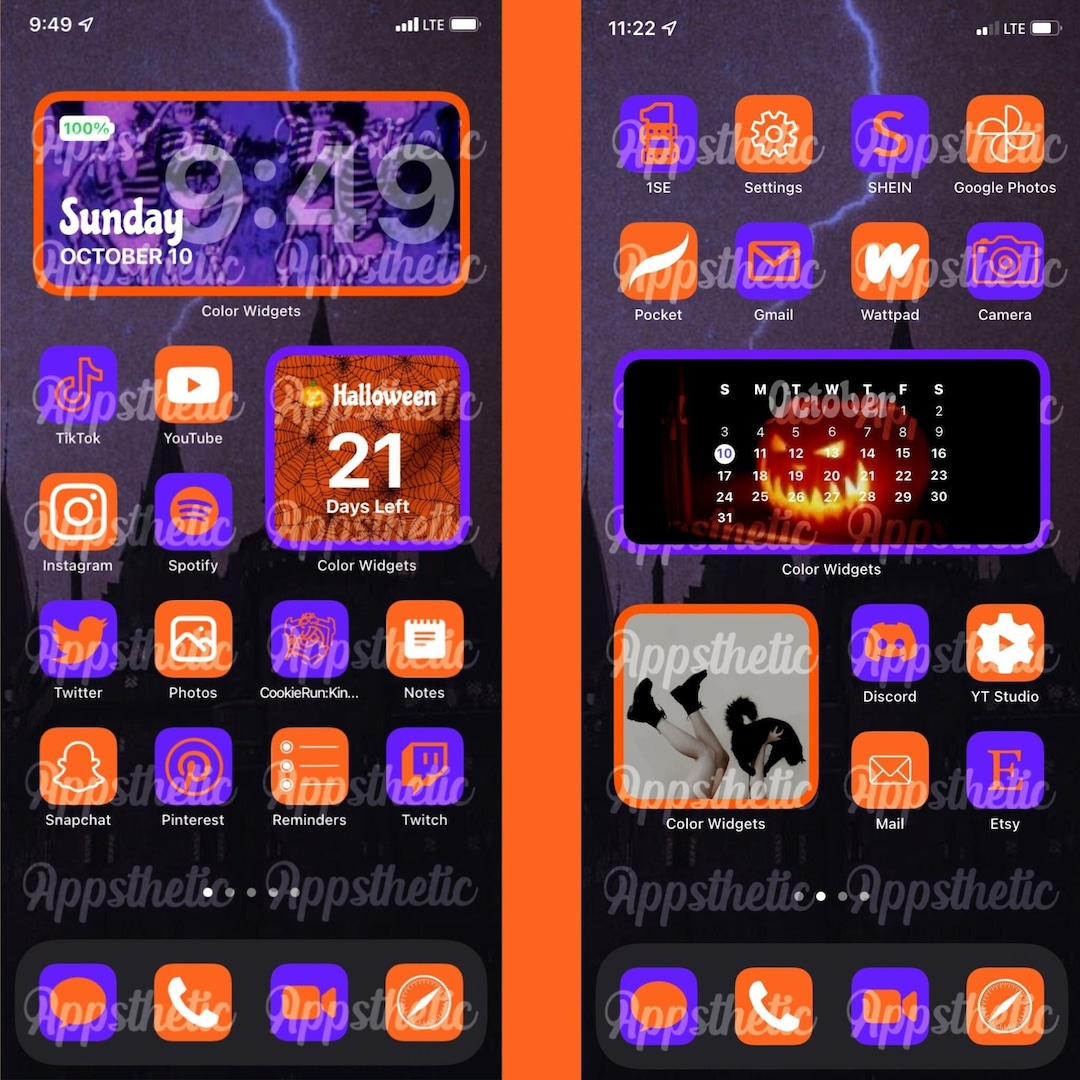The image displays two side-by-side screenshots of a cell phone's home screen, taken at different times. The left screenshot shows the time as 9:49, while the right screenshot displays the time as 11:22. Both screens feature a watermark that reads "Appstatic," indicating the use of a branded theme, likely intended to prevent design theft. 

At the top of the left screenshot, the device status bar shows the date as Sunday, October 10th, with a fully charged battery at 100%. The home screen icons are organized in a horizontal sequence and include TikTok, YouTube, Instagram, Spotify, Color Widgets, Twitter, Photos, Cookie Run: Kingdom, Notes, Snapchat, Pinterest, Reminders, and Twitch. Instead of their usual vibrant iconography, all app icons are themed in blue and orange or orange and white to reflect a Halloween motif.

On the right screenshot, the apps are displayed in rows from left to right and include 1SE, Settings, Shein, Google Photos, Pocket, Gmail, Wattpad, Camera, Calendar, Color Widgets (appearing twice), Discord, YT Studio, Mail, and Etsy. Consistent with the left screenshot, these icons are also designed in the same Halloween-themed blue and orange or orange and white color schemes. 

The consistent branding and thematic color palette suggest the use of an Appstatic design, likely offering specialized and visually cohesive themes for cell phone customization.